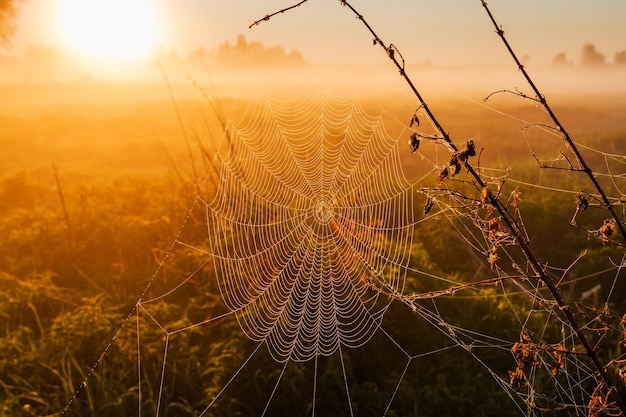This outdoor photograph captures a picturesque scene during either sunrise or sunset, with the sun positioned on the far left, casting a warm, orange glow over the landscape. The background features a gradient sky transitioning from the bright sun to various shades of clouds, extending to the right. Below, the silhouette of trees and foliage of varying sizes frames the horizon. 

In the foreground, a vast field of grass is sprinkled with pink and yellow flowers. Dominating the scene is an intricate spider web, forming a scalloped pattern around the edges and stretching out symmetrically. The web appears gracefully anchored between two prominent twig stems from nearby plants, adding to the delicate beauty of the scene. Thin white lines of the spider web are visibly outlined against the vibrant backdrop, forming a pattern reminiscent of a target. The composition successfully blends the intricate details of the spider web with the serene, sunlit meadow, creating a captivating and tranquil image.